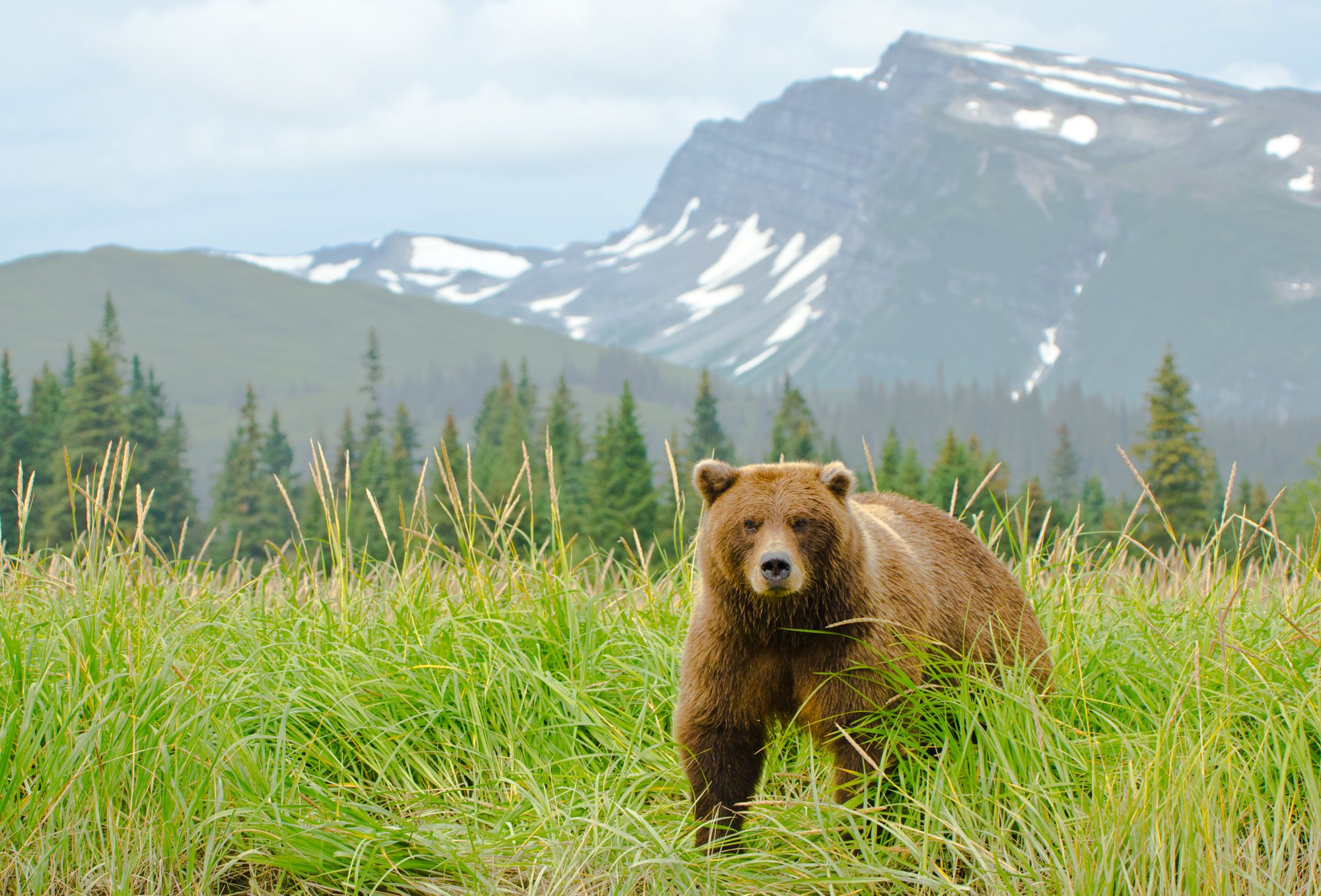This is a detailed photograph of a brown bear standing in a grassy meadow, slightly to the right of the frame and looking directly at the camera. The bear stands amidst tall green and yellow stalks of grass, which are flattened around him as if he had been lying there prior to standing up. His snout is a lighter shade compared to the rest of his body, and only his front legs are visible due to the height of the grass. The backdrop features a row of tall coniferous trees, likely spruce or fir trees, at the middle of the image. Behind the treeline, a hazy mountain range with snow-topped peaks extends across the horizon under a cloudy gray sky. The colors in the photo prominently include the blue sky, dark mountains, green trees and grass, and the brown fur of the bear, which adds to the striking nature of the scene. The overall effect hints at a possibly digitized image, capturing the essence of wildlife in a northern, outdoor setting.